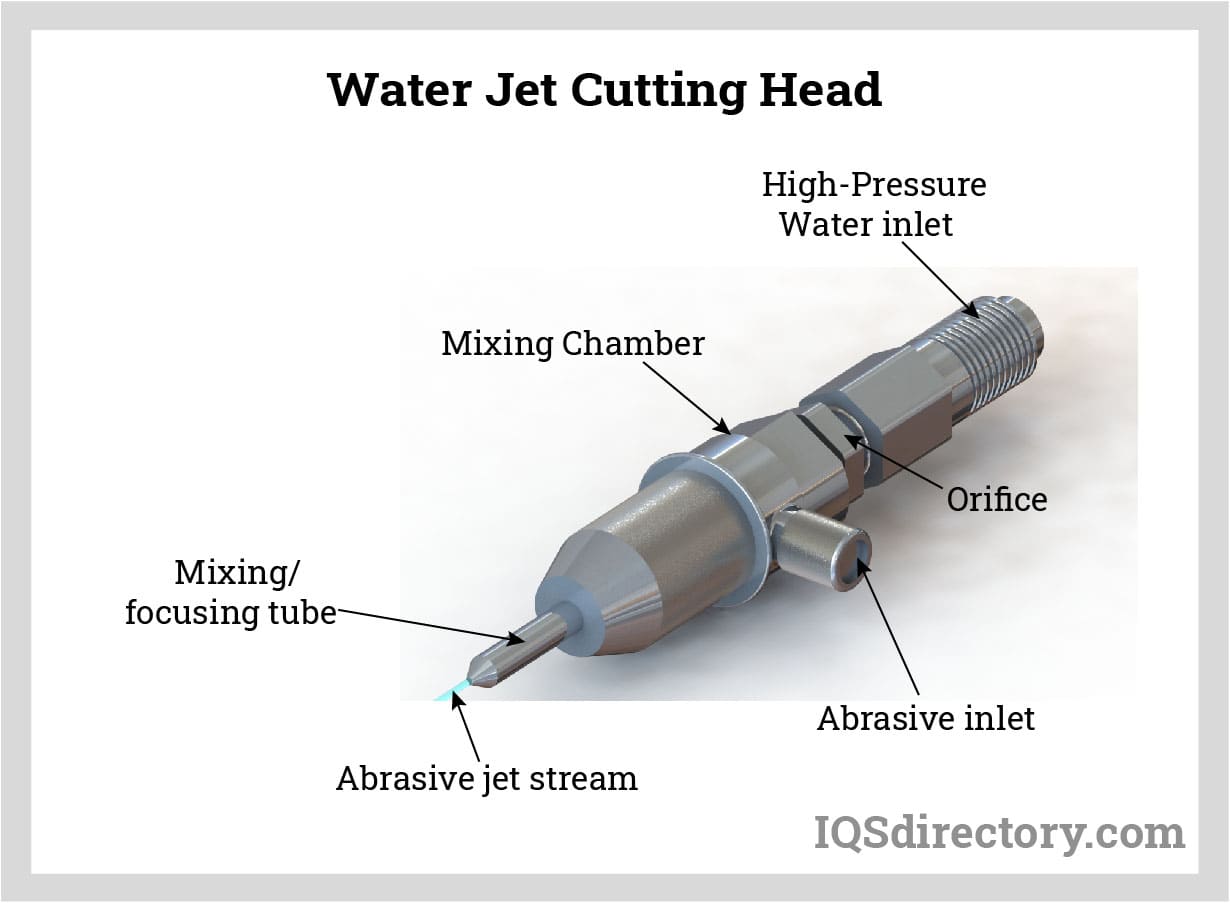The image is a detailed diagram of a water jet cutting head displayed on a white background with a light gray border. At the top of the image, the title "Water Jet Cutting Head" is written in black text. The diagram itself is depicted in dark gray, highlighting different labeled components of the cutting head. Starting from the top right, it indicates the "High Pressure Water Inlet." Moving down, various parts such as the "Orifice," "Mixing Chamber," and "Mixing Focusing Tube" are identified. At the bottom left, the "Abrasive Inlet" is marked, feeding into the "Mixing Chamber." From the "Mixing Focusing Tube," a blue line representing the "Abrasive Jet Stream" emerges. In the bottom right corner, the text "IQSDirectory.com" appears in light gray, serif font. The diagram provides a comprehensive view of the water jet cutting head, illustrating each component's function in the process.